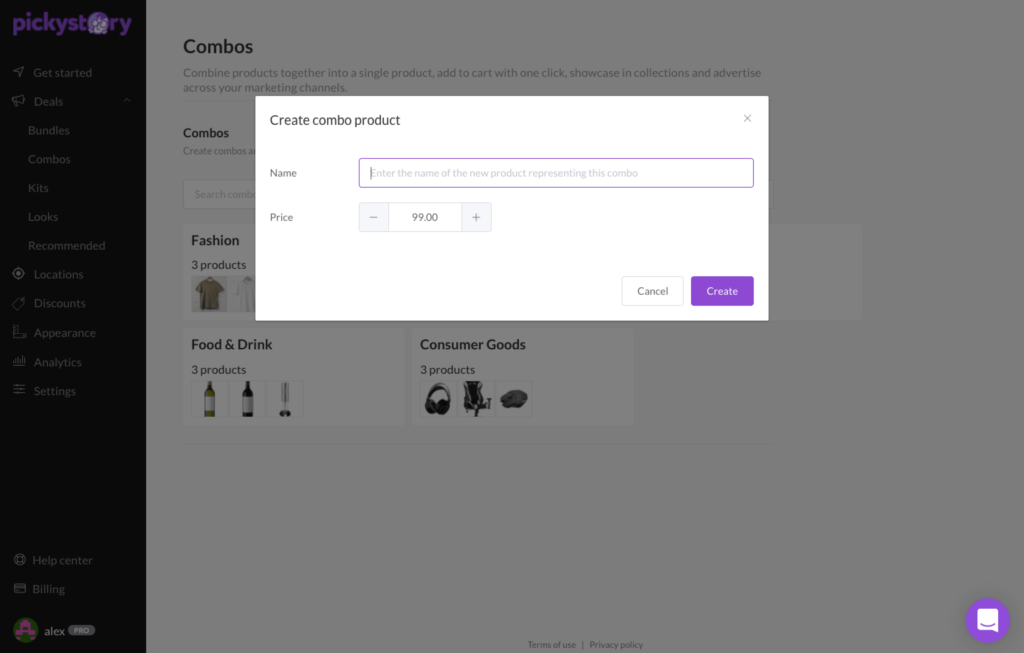In the foreground, a pop-up box takes center stage, inviting users to "Create Combo Product." The box prompts for a product name with a text box showing, "Enter the name of the new product representing this combo." Below, users can adjust the price using a minus and plus sign, currently set at "$99." Two buttons are available: a gray "Cancel" button with dark gray text, and a purple "Create" button with white text.

In the background, the interface of the Picky Story website or app is visible, though slightly blurred. On the left-hand side, a menu contains various options, shown in grayscale. Prominently displayed at the top-center, "Picky Story" is written in purple text within a long black rectangle. Below, product categories are showcased: 

- **Fashion:** Featuring an image of a shirt.
- **Food and Drink:** Displaying two bottles of wine and another unclear item.
- **Consumer Goods:** Showing a gaming chair and a pair of headphones, with the third item indistinguishable.

Above this, a headline reads, "Combo: Combine products together into a single product and add to cart with one click. Showcase collections and advertise across your marketing channels," exemplifying a possible combination like a bottle of wine paired with a wine glass. A search bar is also present, streamlining the navigation for users on the platform.